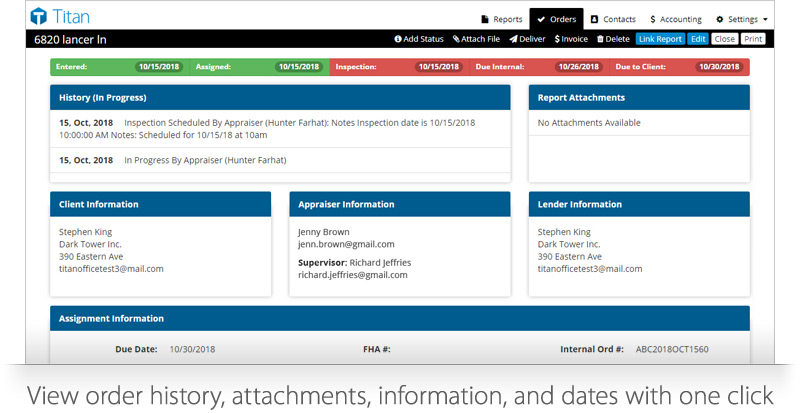This image is a cropped screenshot of the order page from the Titan appraisal app, illustrating the various features and layout of the interface. At the bottom portion, prominent large gray text reads, "View order history, attachments, information, and dates with one click." The screenshot is intended for informational purposes to showcase the versatile features of the app. 

At the top left, the title "Titan" is displayed, indicating the app's branding, followed by an indication that the user is on the "Orders" tab. Directly beneath, several sections are outlined, including "History and Progress," "Client Information," "Appraiser Information," and "Lender Information." Further down, another section labeled "Assignment Information" is cropped out of the screenshot.

A green bar situated at the top left shows the word "Entered" on the left side, followed by a date, and the term "Assigned" is listed to the right with another corresponding date. Adjacent to this section, a large red bar stretches to the right side of the page with the word "Inspections" and a date listed next to it. Below this, additional dates are provided under headers "Due Internal" and "Due to Client," each tagged with their respective deadlines.

This organized layout offers a comprehensive look at the systematic and user-friendly design of the Titan appraisal app, highlighting key features and functionalities useful for managing appraisal orders.